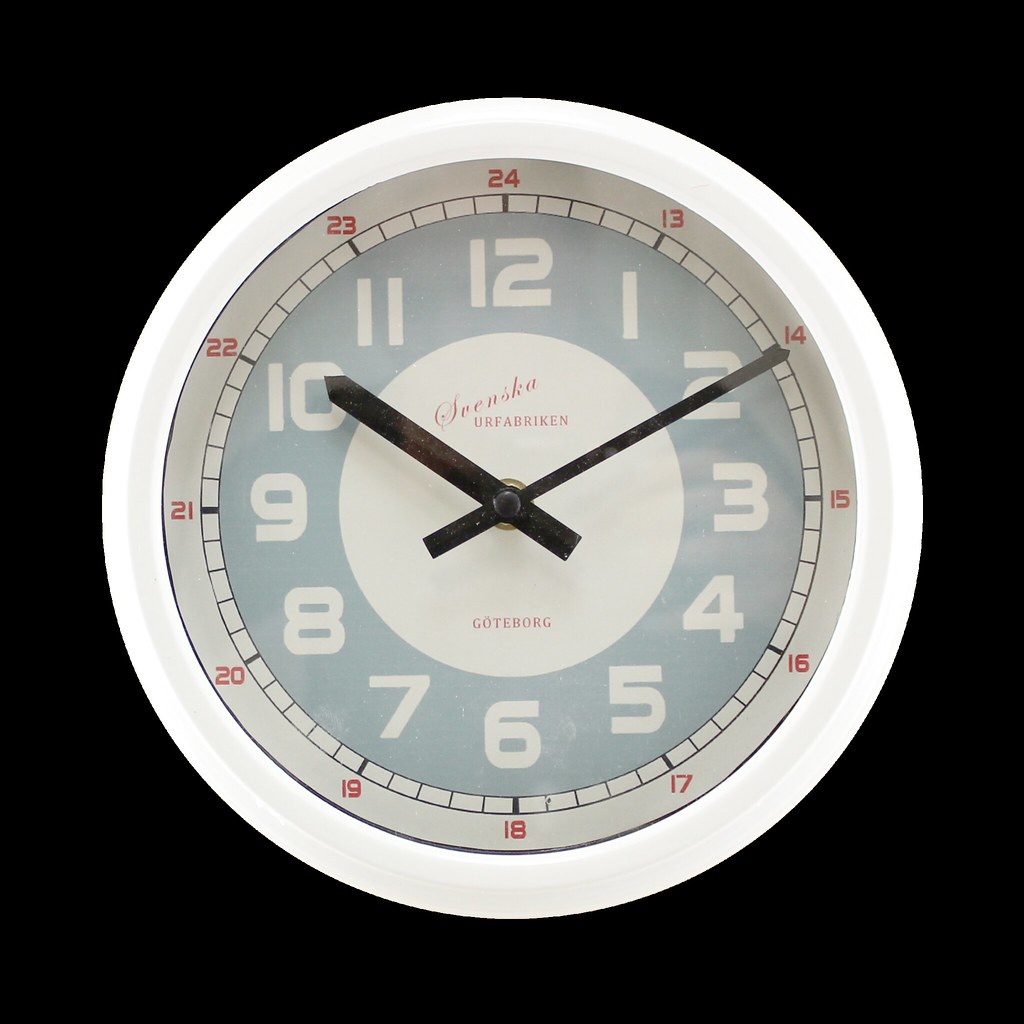This image depicts a detailed, abstract, computer-generated wall clock with a distinctive appearance and a striking Art Deco style. The clock features a central white circle from which basic black hour and minute hands (currently showing the time as 10:10) originate. The face contains normal digits (1 to 12) in white on a light blue ring. Surrounding this main circle is an intricate, narrow white rim with additional numbers marking military time (from 13 to 24) in red, located just outside the primary hour markers. The clock is mounted against an entirely black background, enhancing the contrast and making the clock's design stand out prominently. Adding to the artistic touch, the center of the clock includes text in Swedish, "Svenska Örfabriken Göteborg," signifying its origin or stylistic inspiration from Sweden, particularly Göteborg.